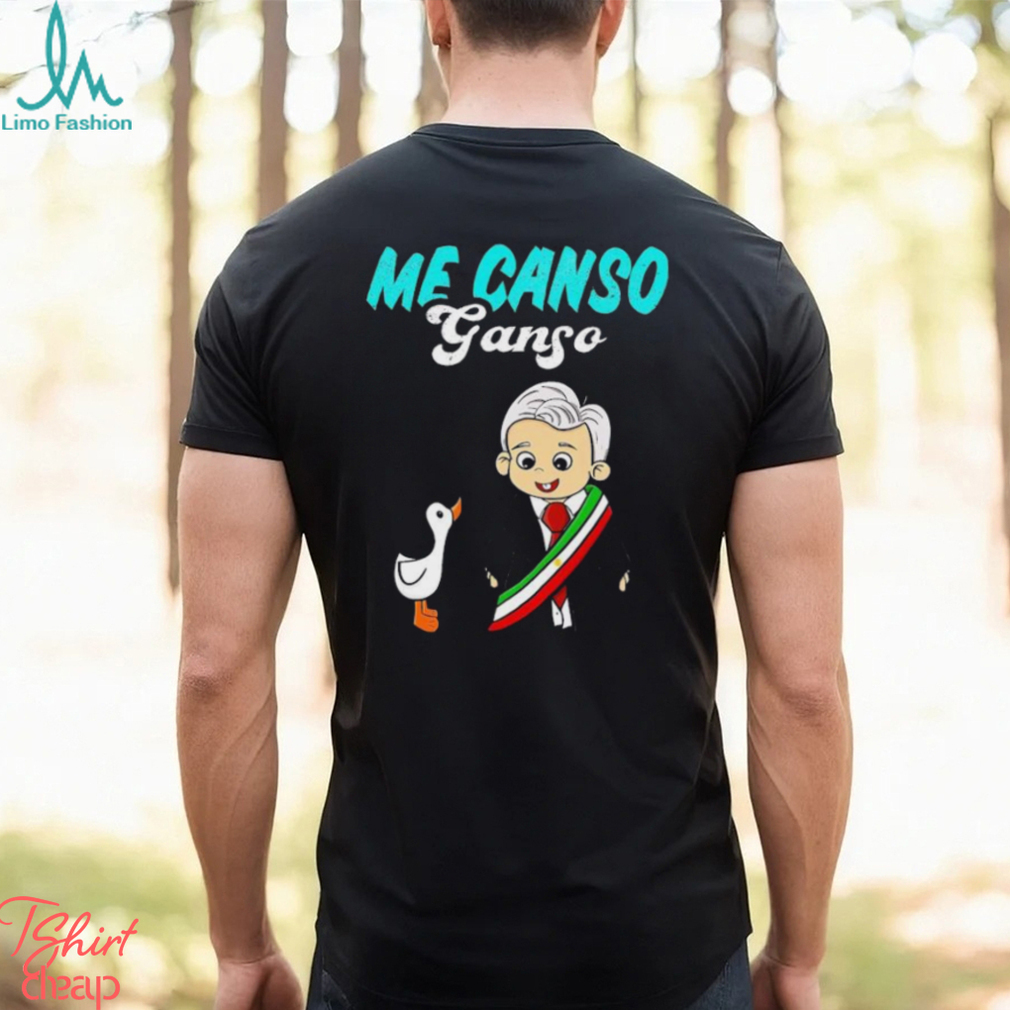In this advertisement for a fashion brand, a man stands in a forest scene, his back facing the camera. He is wearing a snug, black t-shirt that prominently displays various designs and text. The t-shirt's upper portion features the brand name "Limo Fashion" in green cursive letters, accompanied by a logo in the upper left corner. Just below that, in bright blue letters, it reads "ME CANSO." Further down, in white letters, the word "G-A-N-G-O" is displayed. Underneath the text, there are two distinct graphics: a cartoon duck facing right and a figure of a man with white hair, dressed in a suit and red tie, accented with a green, white, and red sash — possibly indicating an Italian-themed design. The lower left corner of the shirt highlights in pink the product type: "T-shirt, CHEAP." The background is softly focused, revealing faint tree trunks and a hint of grass, adding a touch of nature to the scene. This detailed and eye-catching design emphasizes the unique and stylish aspects of the brand's fashion-forward t-shirts.